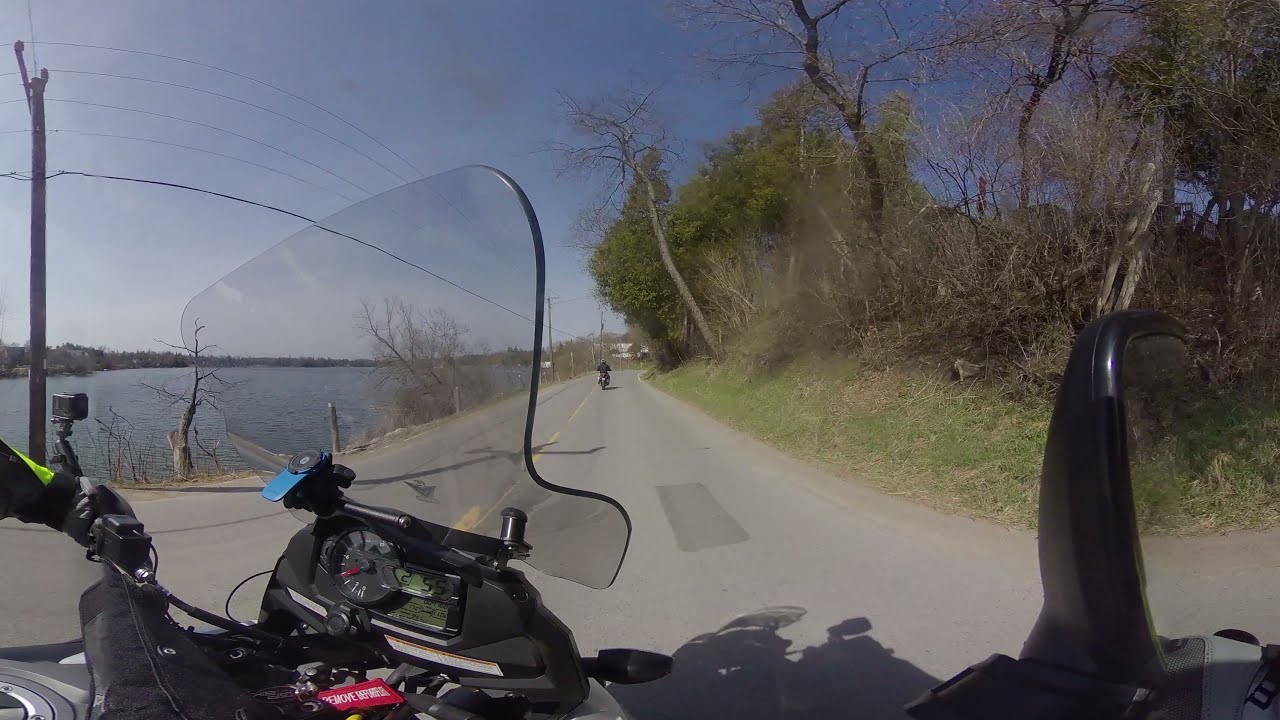In this image, taken from the perspective of someone riding a motorcycle, the viewer can see various detailed elements, emphasizing the scene’s rural, riverside setting. At the forefront, the motorcycle’s black dashboard is visible, featuring its controls, speedometer, and a prominent plastic windshield. A hand donning a black leather glove and a black sleeve with lime green accents grips the left handlebar. To the right, a reflective mirror can be seen.

Ahead, the two-lane paved road with yellow dotted lines stretches out, dividing the image. Further up the road, another motorcyclist rides in the same direction. On the left side of the road, brushy areas and utility poles with multiple horizontal wires span across the scene. The shoreline reveals a large river, with trees lining the horizon on the opposite bank. On the right side of the road, there is a grassy embankment with overgrown vegetation, including shaggy, smaller, and some evergreen trees. The overall setting suggests a scenic, rural ride alongside a river.